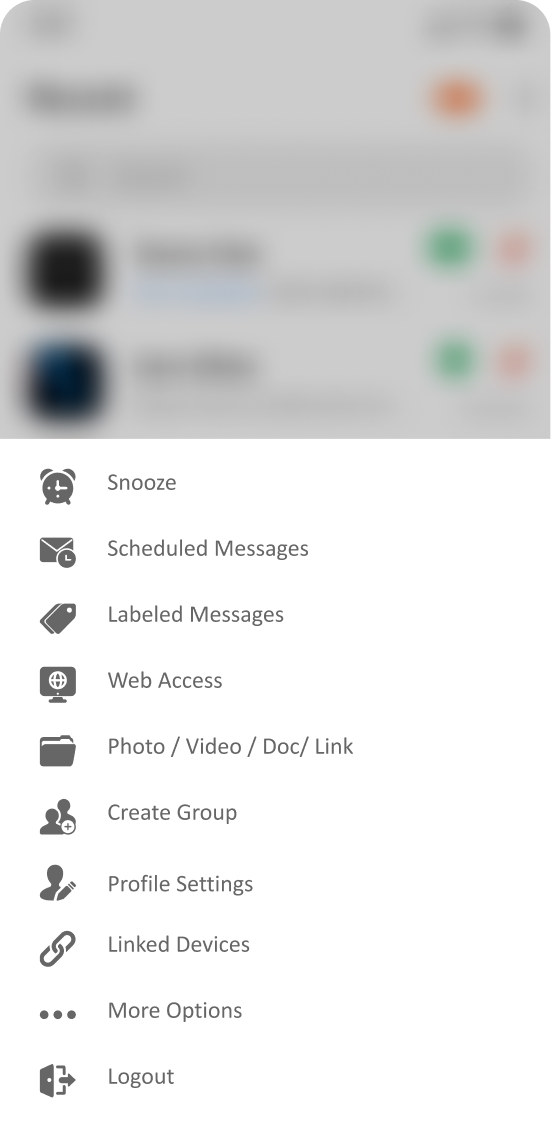The image features a gray background with two blurry black spots on the left side, and possible text on the right, though the text is difficult to discern. There are several colorful icons: an orange circle, two green circles, and two pink circles. Blue text is also visible in the image. Below this section, there is a list of icons accompanied by descriptions. The icons and descriptions, from top to bottom, are as follows:

1. A snooze icon labeled "Snooze."
2. An envelope icon labeled "Schedule Messages."
3. A tag icon labeled "Labeled Messages."
4. A globe icon labeled "Web Access."
5. An icon labeled "Photo/Video/Doc/Link."
6. An icon labeled "Create Group."
7. An icon labeled "Profile Settings."
8. An icon labeled "Link Devices."
9. An icon labeled "More Options."
10. A door icon labeled "Log Out."